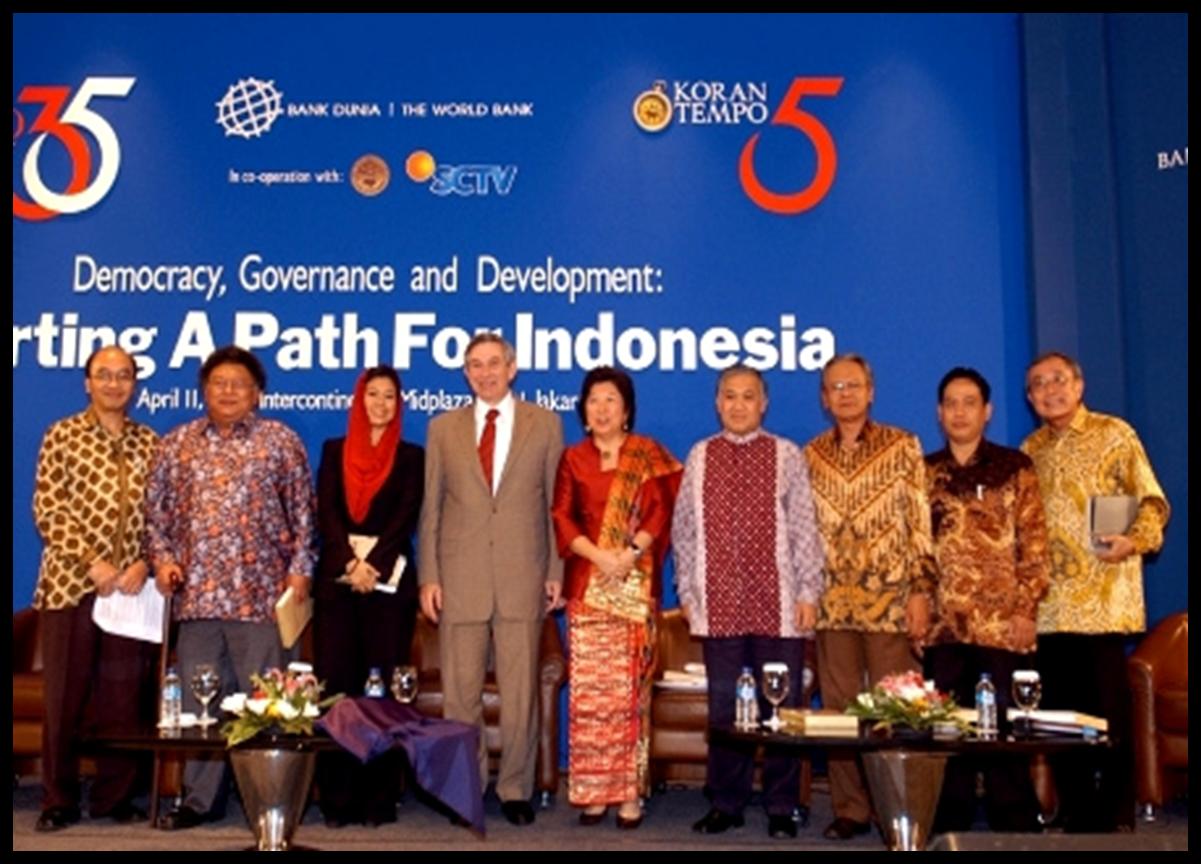The photograph features nine individuals, including both men and women, who appear to be of Korean and possibly Indonesian descent, judging by their attire and the content of the sign behind them. They are gathered in front of a brightly colored blue backdrop, adorned with bold white and red letters that partially read "Democracy, Governance, and Development: A Path for Indonesia" beneath a larger, partially cropped title that includes "Koren Tempo." The group is dressed in an assortment of traditional and modern clothing. Many wear colorful and intricate garments with patterns in gold, yellow, brown, and red; one woman stands out in a long orange and gold skirt with a scarf draped over her shoulder, while another wears a striking red headscarf. At the center of the group, a man dressed in a tan suit and red tie is notably different, possibly hinting at a diverse, multicultural event. In front of them, a small table holds drinks and possibly food, adding to the ambiance of what seems to be a formal event, such as a conference or award ceremony. The mix of traditional attire and formal wear, combined with the signage, suggests a significant cultural or governmental occasion.